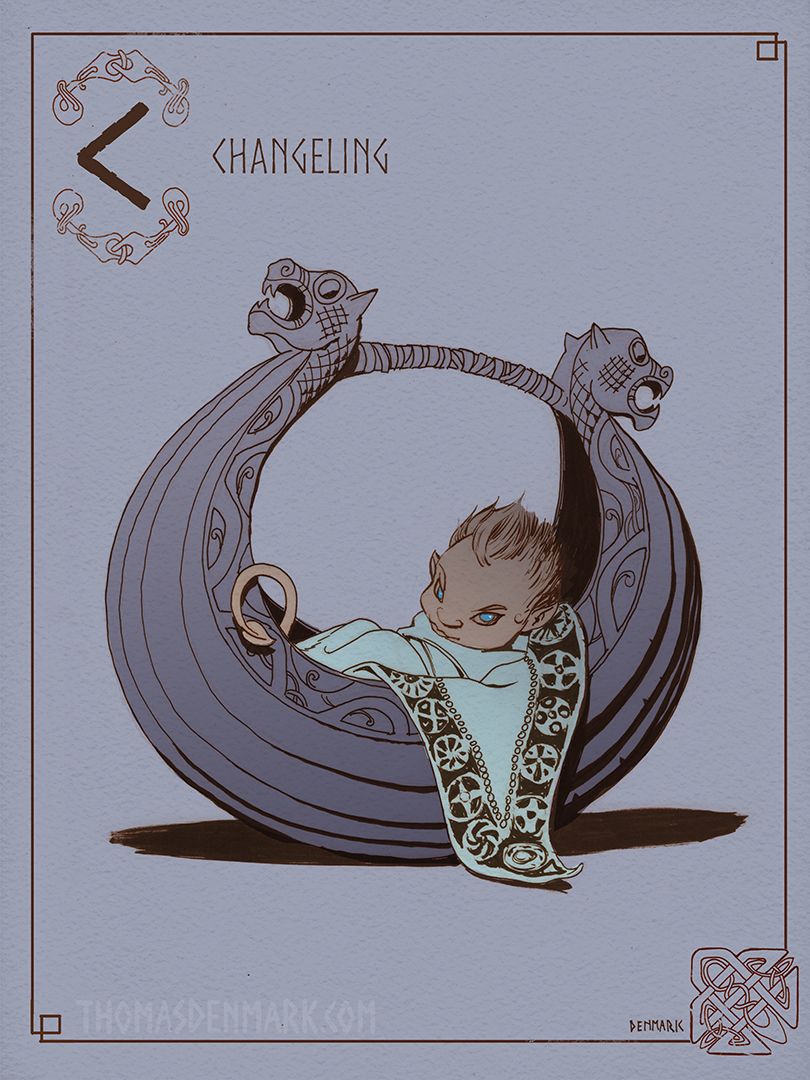The image depicts a card or drawing featuring a fantastical baby creature, prominently labeled "Changeling" at the top. The background is a muted blend of purplish, bluish, and gray tones, adding a mysterious aura to the scene. This card, possibly used for tarot or storytelling, showcases intricate details: a dark gold border with design elements on the lower right side. The central figure is a baby with striking, icy blue gemstone-like eyes and elongated, pointy ears suggesting elf-like or otherworldly origins. Its hair is medium blonde and spiky. The baby is lying in a non-woven basket, which has an elaborate design featuring two dragon heads forming the handles. Additionally, symbols adorn the upper and lower sections of the card. The artist's signature, "ThomasDenmark.com," appears in the lower left corner, while "Denmark" is inscribed on the lower right. The overall composition and lighting, including a subtle blue blanket and the gray coloring of the basket, give the entire card a fantastical and eerie appearance, emphasizing its mythical theme.